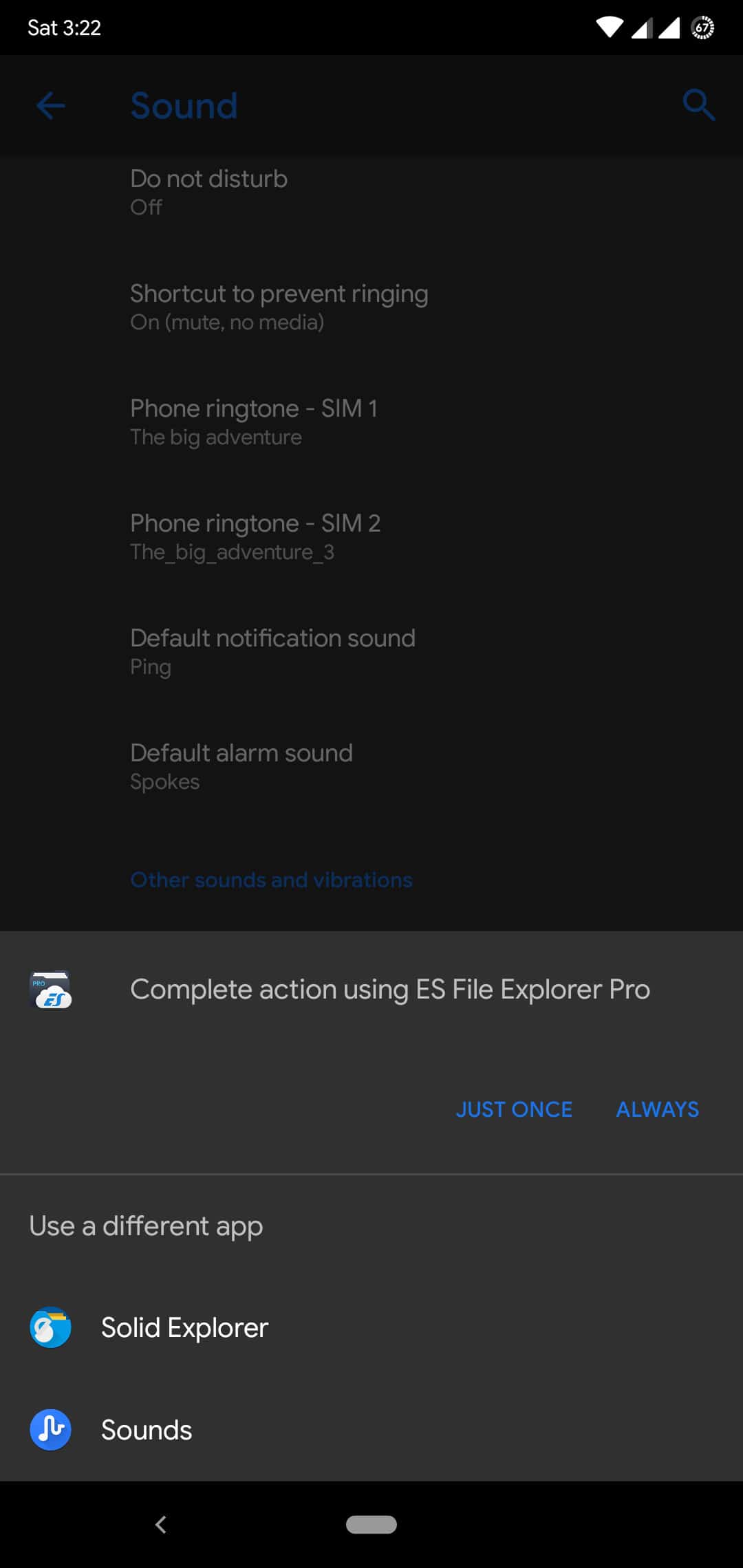### Detailed Caption

This image captures a screenshot from an Android device displaying the settings related to sound and notifications. 

- **Top Bar Details:**
  - **Date & Time:** The status bar indicates it is Saturday, the 2nd of March.
  - **Connectivity & Battery:** On the top right corner, a full Wi-Fi symbol represented by two triangles shows stable connectivity, and the battery icon reveals the device is at 67% charge.

- **Sound & Notifications Settings:**
  - **Current Page Title:** The settings page is focused on sound and notifications.
  - **Do Not Disturb:** 'Do Not Disturb' mode is switched off.
  - **Shortcut Options:**
    - **Prevent Ringing:** There is a shortcut to prevent ringing, and it is currently set to 'Mute'.
  - **Phone Ringtones:** 
    - **SIM 1:** The ringtone is named 'The Big Adventure'.
    - **SIM 2:** The ringtone is labeled 'The Big Adventure_3'.
  - **Notification Sound:** The default notification sound is set to 'Ping'.
  - **Alarm Sound:** The default alarm sound is 'Spokes'.
  - **Additional Settings:** A clickable option labeled 'Other sounds and vibrations' is highlighted in blue.

- **Popup Screen:**
  - **Action Selection:** The user has interacted with an option prompting a popup titled 'Complete action using ES File Explorer Pro' against a dark gray background.
  - **Action Choices:** The options provided are 'Just Once' and 'Always'. Below a gray dividing line, another selection specifies 'Use it for app', with choices being 'Solid Explorer' or 'Sounds'.

- **Navigation:**
  - **Bottom Navigation:** Visible navigation buttons at the bottom include a home button and a back arrow pointing left.

This detailed description covers all elements and interactions visible in the screenshot, providing a comprehensive overview of the content displayed on the device.